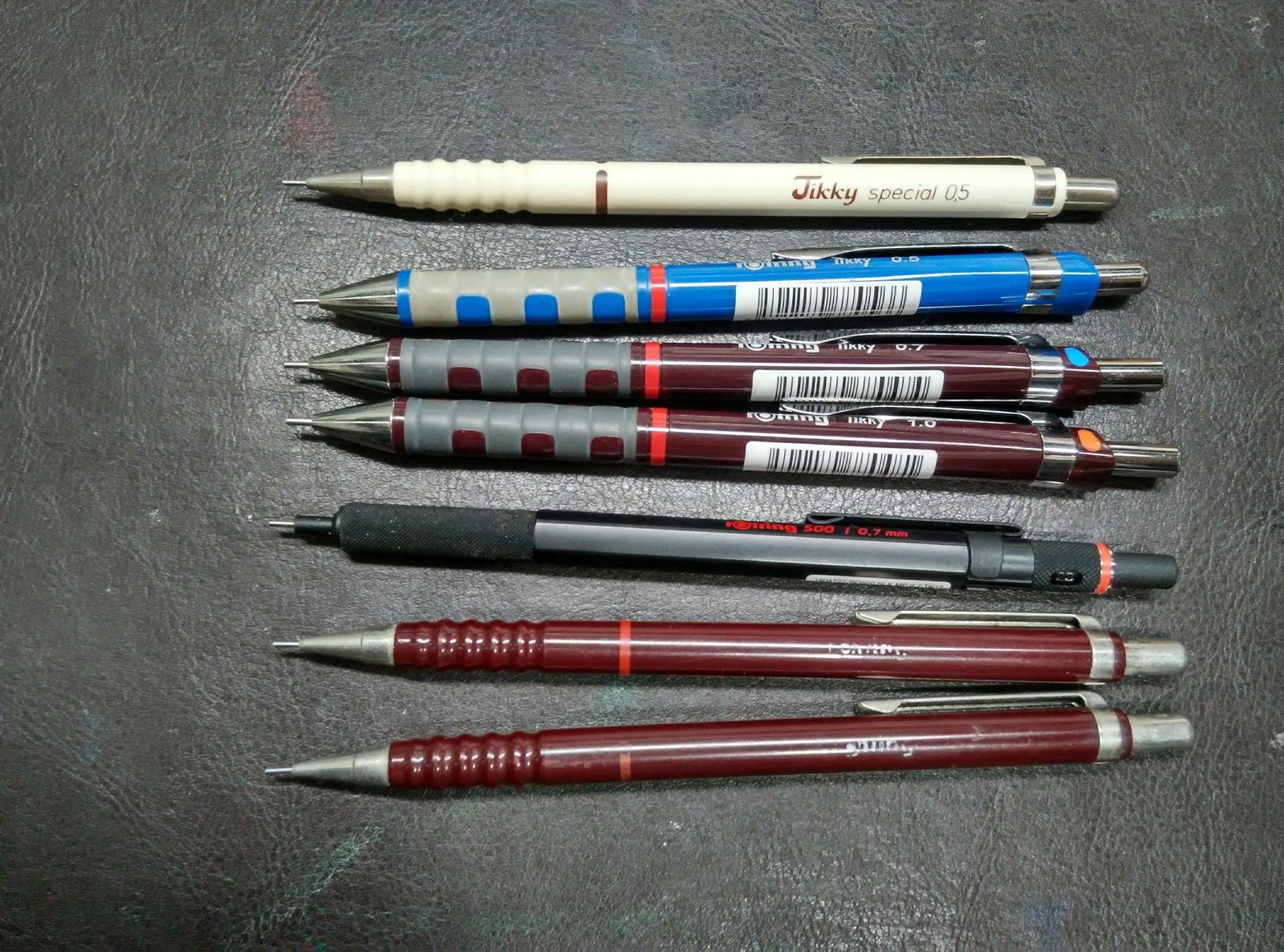In the image, seven pens are arranged horizontally on a grey leather-like background that appears slightly brighter in the center. The surface, possibly a notebook or journal cover, features faint streaks of green, blue, and red. 

The top pen is white with a red stripe and text reading "JIKKY Special 0.5," featuring silver accents and a clip. The second pen is blue with a silver tip and clip, a red stripe, a barcode, and small, illegible letters at the top. The third and fourth pens are maroon with gray grips, silver clips, and barcodes; the third has a blue spot at the top, while the fourth has an orange spot. The fifth pen is black with light and dark grey elements, transitioning from lighter to darker shades towards the bottom, and ending in a black-and-silver tip. The sixth and seventh pens are maroon with silver clips and accents, and while similar in design, the seventh has a slightly different stripe pattern near the top. All pens have comfort grips, and their varied colors and lengths provide a visual contrast against the textured background.